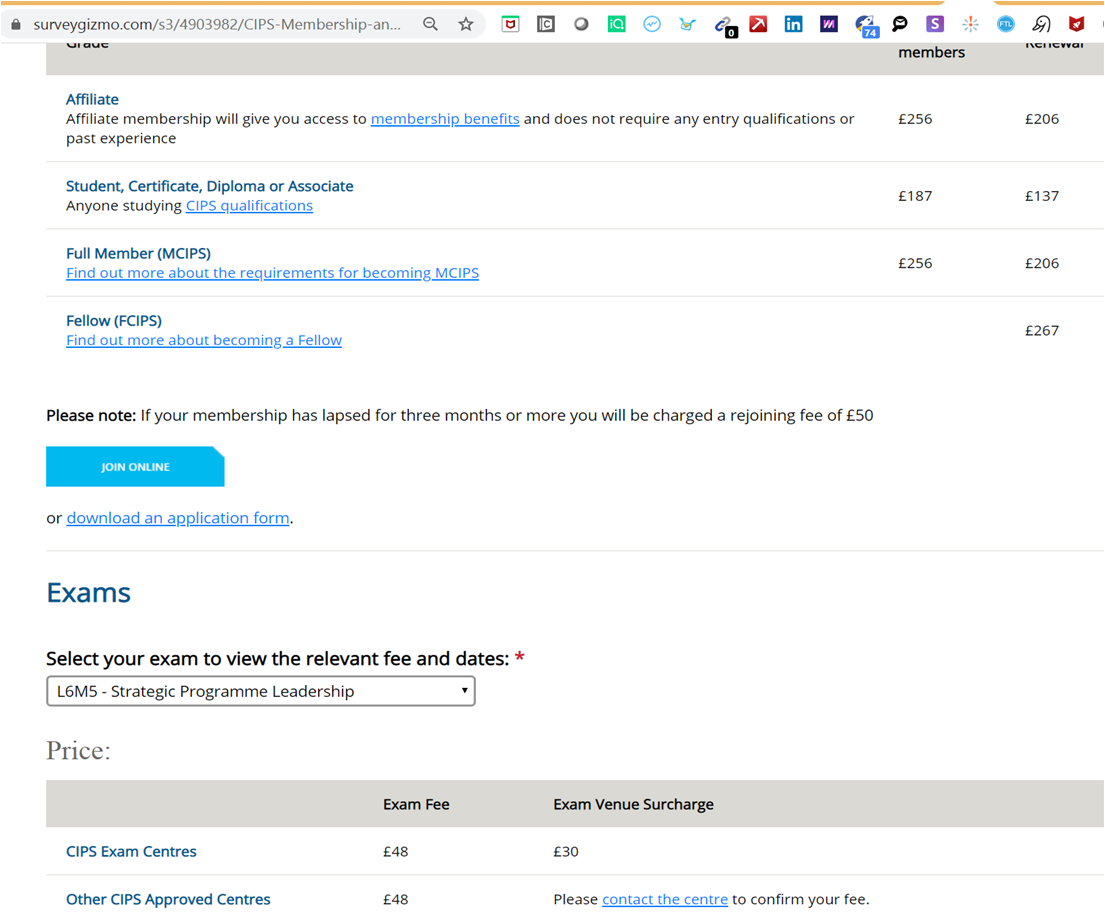**Caption:**
The image features a screenshot of a webpage from SurveyGizmo.com against a white background. The screenshot contains detailed information about various membership types and associated benefits. It announces that an affiliate membership provides access to membership benefits without requiring any entry qualifications or past experience. The types of memberships listed include Student, Certificate, Diploma, Associate, Full Member, and Fellow. A notable statement mentions that if a membership has lapsed for three months or more, a rejoining fee of £50 will be incurred. At the bottom of the webpage, there's a blue rectangular "Join Online" button. Below this, the text instructs users to "select your exam to view the relevant fee and dates." An exam titled "L6M5 Strategic Program Leadership" is noted, with exam fees detailed as £49 for the CIPS exam center and a £30 exam venue surcharge.